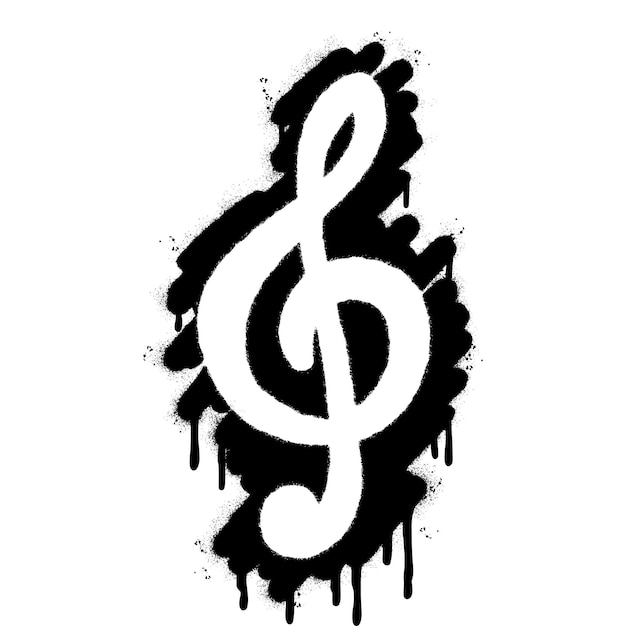The image is a detailed illustration or painting featuring a special character, an ampersand, which is centrally positioned. The ampersand, shaped like an 'S', is painted in a large, blocky, and smooth white form with flowing curves. This white ampersand stands out against a black background, which exhibits a textured, dripping paint effect. The background features diagonal black streaks that drift from the bottom right to the top left, giving a sense of movement and dynamism. These streaks appear as though they are cascading downwards, with individual drips of black liquid hanging from the ends. The entire scene, with its sharply contrasting elements, is set against a plain white backdrop. The overall style of the piece combines the complexity of a painting with a stark black and white color scheme, creating a striking and evocative visual.